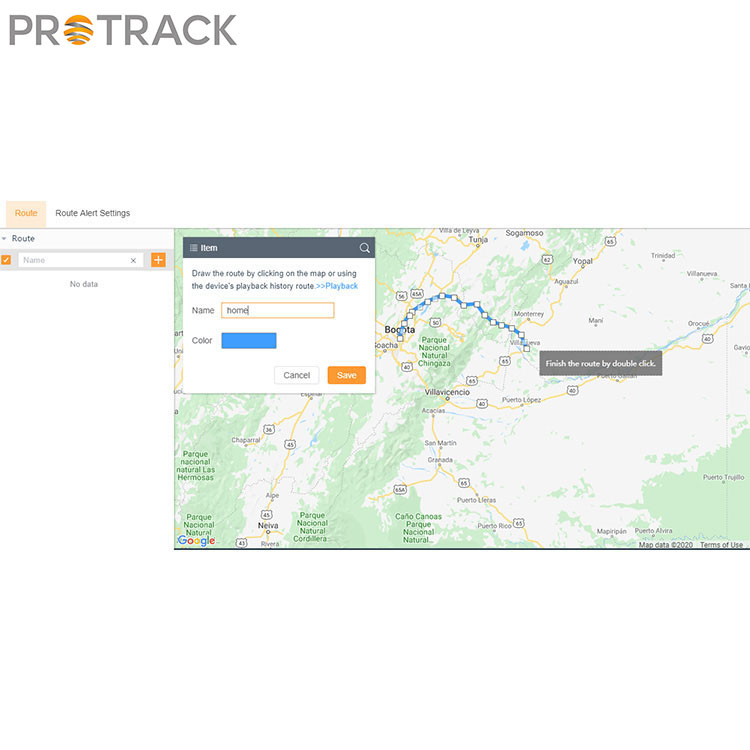**Caption:**

The image, categorized under 'Websites', depicts a small, intricate map interface focused on route management, resembling Google Maps. In the top right corner, the word "Route" is highlighted, accompanied by "Route Alert Settings" positioned nearby. Below, the interface displays an orange check mark next to "Route" within an active white box. This section includes the labels "Name" and "No Data", and instructs users to "Draw the route by clicking on the map or using the device's playback history route". 

An option to initiate playback is offered through clickable text that reads "Playback". Further details reveal the route name is set as "Home" and the chosen route color is blue. The central map prominently focuses on Bogota, displaying a network of blue lines and dots forming a plotted route beginning in Bogota. To finalize the route, users are prompted to "finish the route by double click". Although the image quality restricts further enlargement, it hints at additional detailed elements scattered across the map.